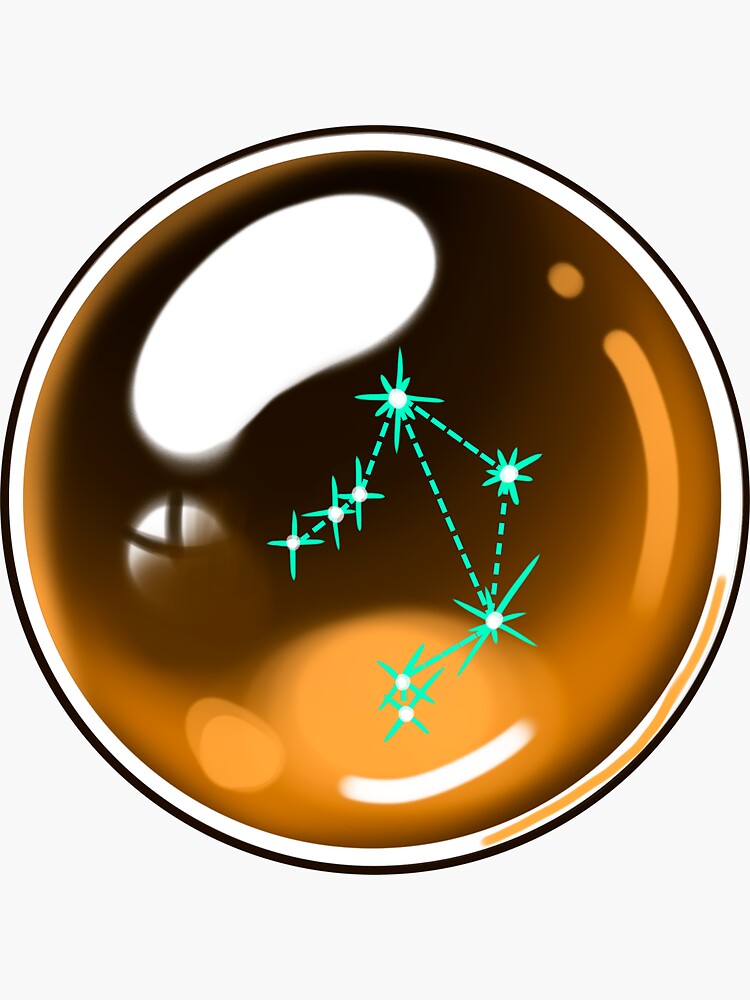This is a detailed depiction of a digital 3D art image, resembling a glossy orb or sphere, possibly akin to a sticker or logo. The image features a multi-layered circular design starting with a thin black outer ring, followed by a thicker white ring. On the bottom right segment of the white ring, an orange stripe pierces through, adding a striking accent. Encased within these outer rings, the core of the orb presents a gradient blend of tan, brown, and black colors, with the bottom half predominantly glossy orange and black.

The top-left section of the orb showcases a prominent white, footprint-shaped smudge, symbolizing the shininess of the object. Below this, there is a smaller, partially gray-outlined white circle resembling a stylized 'X,' reminiscent of the X-Box logo. The bottom right of the orb features a distinct orange blob, enhancing the overall vibrancy.

Central to the design is an intricate constellation of turquoise stars, interconnected by delicate dotted lines. These stars, each featuring a white center, are meticulously placed and connected, creating a visually appealing pattern that stands out against the mocha tan background. The stars and their connecting lines give the image a celestial ambiance, almost suggesting a map of the night sky.

Overall, the composition of black, white, brown, tan, orange, and turquoise elements, combined with the glossy texture and precise highlights, gives this orb a lifelike, reflective quality, effectively capturing attention and stimulating curiosity.